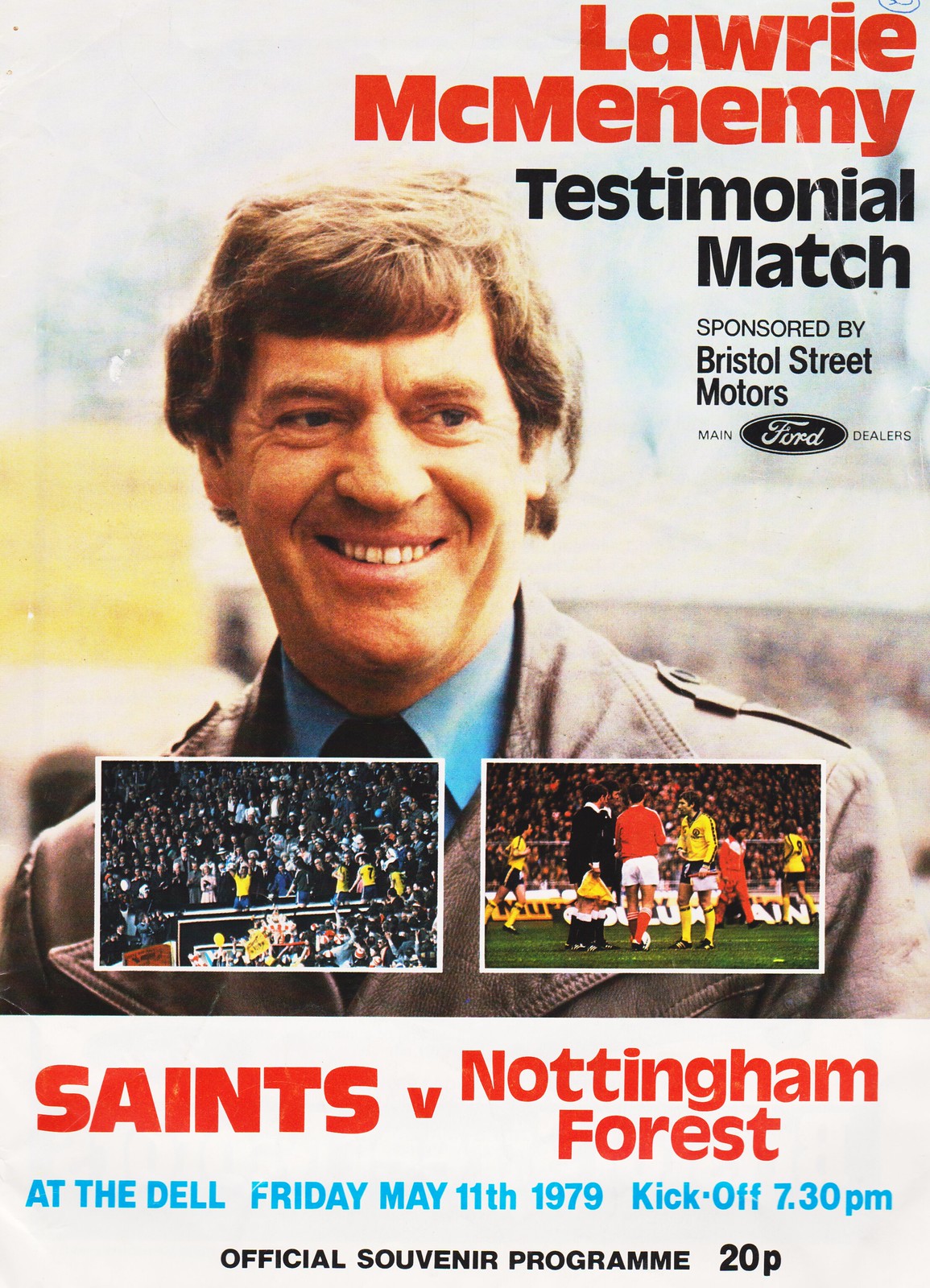This image appears to be an advertisement for an upcoming football testimonial match from 1979, specifically displayed as a colorful program or magazine page. At the top, it prominently features the text "Laurie McMenemy Testimonial Match, sponsored by Bristol Street Motors, main Ford dealers." A smiling man in his late 40s with brown hair, blue eyes, and wearing a trench coat, blue shirt, and tie is pictured, identified as Laurie McMenemy. Below his image, there are two smaller photos: one showing a stadium filled with fans and the other depicting a scene from a football match. In the match photo, players are seen in yellow and black uniforms and red and white uniforms, possibly involved in a discussion with referees. The upcoming game is between the Saints and Nottingham Forest, scheduled to be played at the Dell on Friday, May 11th, 1979, with a kickoff at 7:30 p.m. The page notes that it is the official souvenir program, priced at 20p.